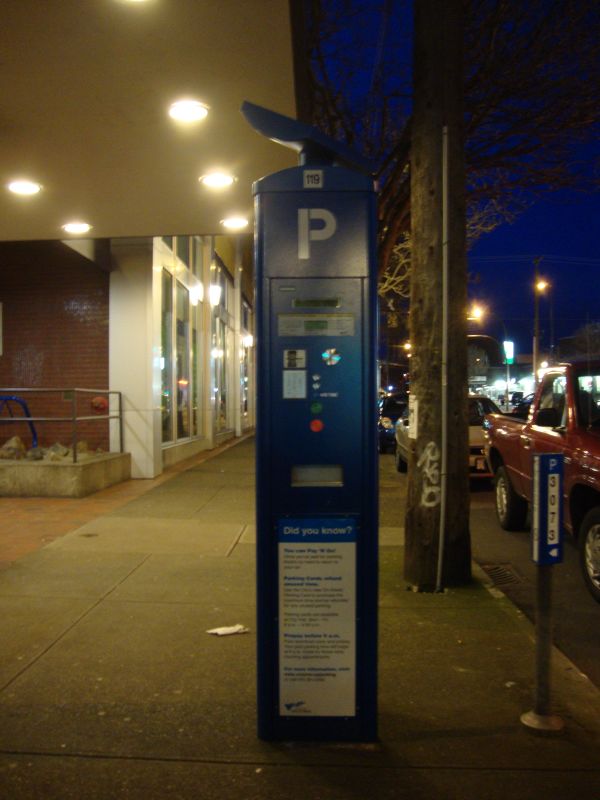This color photograph, in a vertical rectangle or portrait orientation, depicts a nighttime city street scene under a rich, dark blue sky. On the left, a brick building with white window frames and plate glass windows extends into the background, featuring an awning or overhang from which tungsten lights illuminate the scene. In the center of the sidewalk stands a tall, dark blue parking meter with a prominent white "P" at the top. This meter features slots, buttons, and a display terminal for payment, along with a detailed informational sign at its base. To the right, cars, including a red pickup truck, are parked along the street, with streetlights and brightly lit street signs in the distance. Additionally, there's a small metal post marked with the number 3073. A tree with low-down graffiti also stands nearby, adding an unfortunate blemish to the otherwise orderly streetscape. Litter is scattered on the sidewalk, reflecting the wear of a bustling urban environment.